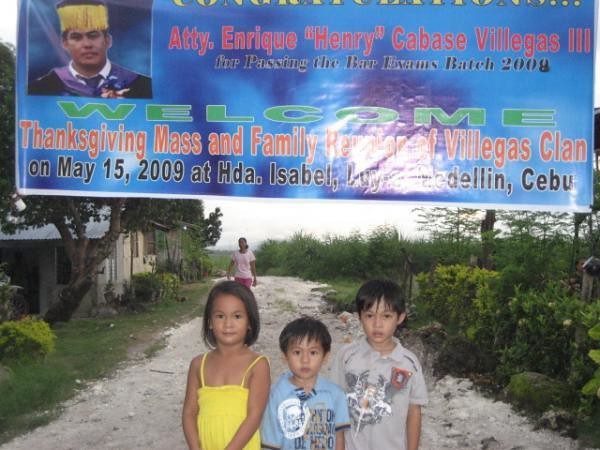The image depicts a scene of three young children standing on a light gray dirt pathway in a village. Above them hangs a blue banner that reads, "Welcome Thanksgiving Mass and Family Villegas Clan on May 15, 2009 at HDA Isabel," suggesting an event or gathering. The children face the camera with somber expressions. On the left is a girl dressed in a yellow tank top, in the middle stands a boy in a blue polo shirt with some writing on it, and on the far right is a boy in a gray short-sleeved polo shirt. Behind them, a woman wearing a pink shirt and pink pants is walking towards the children. To the far left of the image, there is an older tin-roof house, partially obscured by a tree and several green shrubs. The sky above is mostly white and overcast.